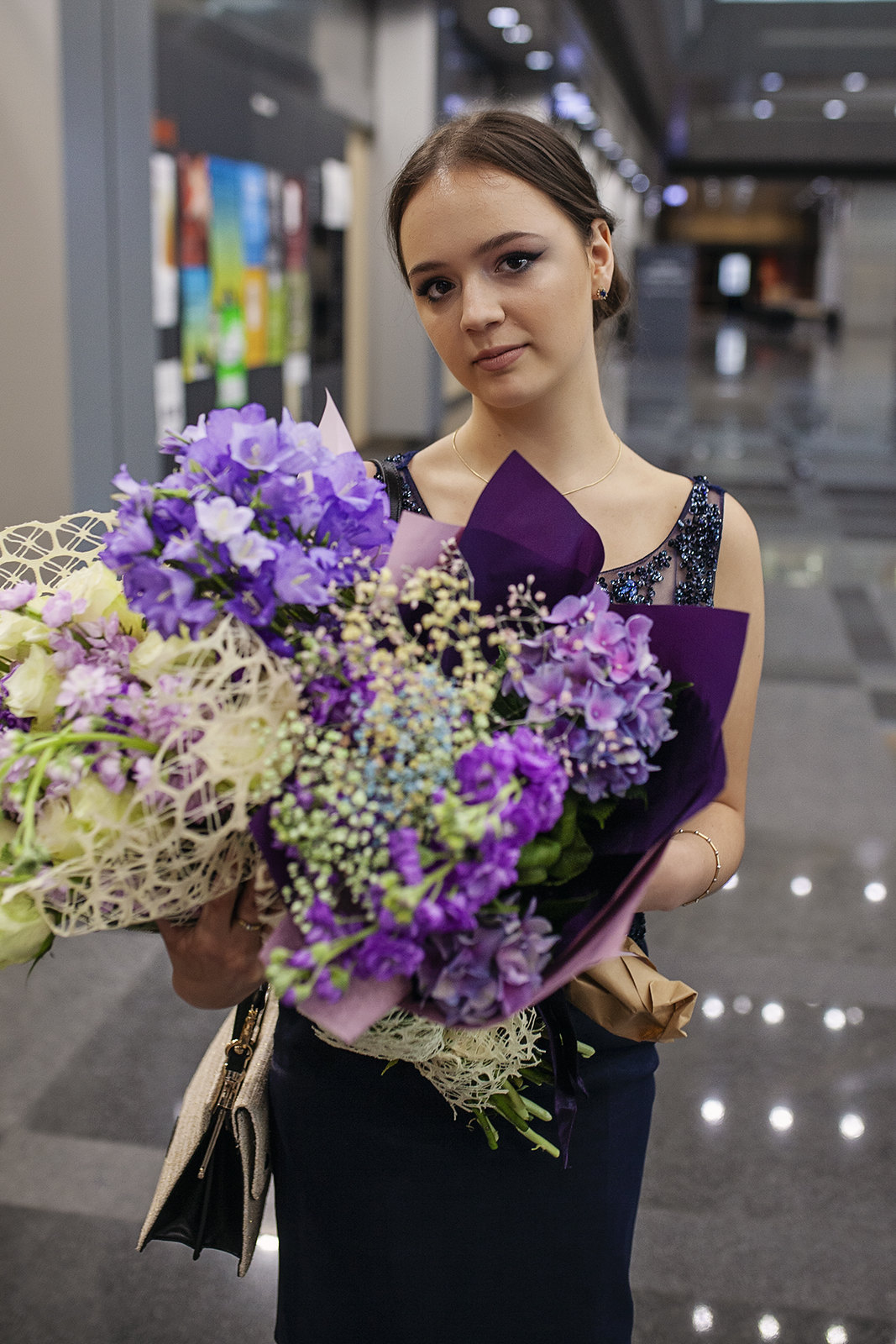In this portrait-oriented photograph, a young woman, likely in her late teens or early twenties, stands centrally, showcasing her elegant style. She is dressed in a dark blue, sleeveless formal dress adorned with intricate beading at the top. Her auburn hair is neatly pulled back, and her makeup is meticulously done, highlighting her eyes with eyeliner. She holds three distinct bundles of flowers in front of her, featuring a mix of purple, yellow, and pink blooms. The flowers are wrapped differently: one in purple paper, another in white lace, and the third appears unwrapped. A cream-colored purse hangs elegantly off her hip. The indoor setting resembles a shopping mall or a similarly well-lit environment, with blurry background elements hinting at shops and shiny stone floors. The walkway she stands on appears to be concrete, silver, or gray in color, contributing to the photograph's polished aesthetic.